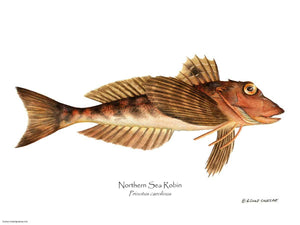The image is a vintage artistic rendering of a "Northern Sea Robin," as indicated by the clear black text beneath the fish, along with some additional, harder-to-read writing and an artist's signature. Set against a stark white background, the fish is depicted horizontally and appears very antiquated, possibly from an old book or poster. Its body color transitions from a deep orange-red to brown, adorned with black tiger-like stripes along its back, tail, and part of its fins, which are golden with black accents. It has a dark orange head with a slightly open mouth, sharp and pointed, and large, round amber eyes with black pupils and green outer edges. The fish boasts a long dorsal fin running along its back and an inverted fin under its belly, with smaller pectoral fins near its neck and two lateral fins visible towards the sides. Adding a whimsical touch, three whisker-like structures extend from beneath its chin. The detailed and colored penciling gives the fish a realistic yet artistic appearance, capturing the essence of an ancient sea creature meticulously.